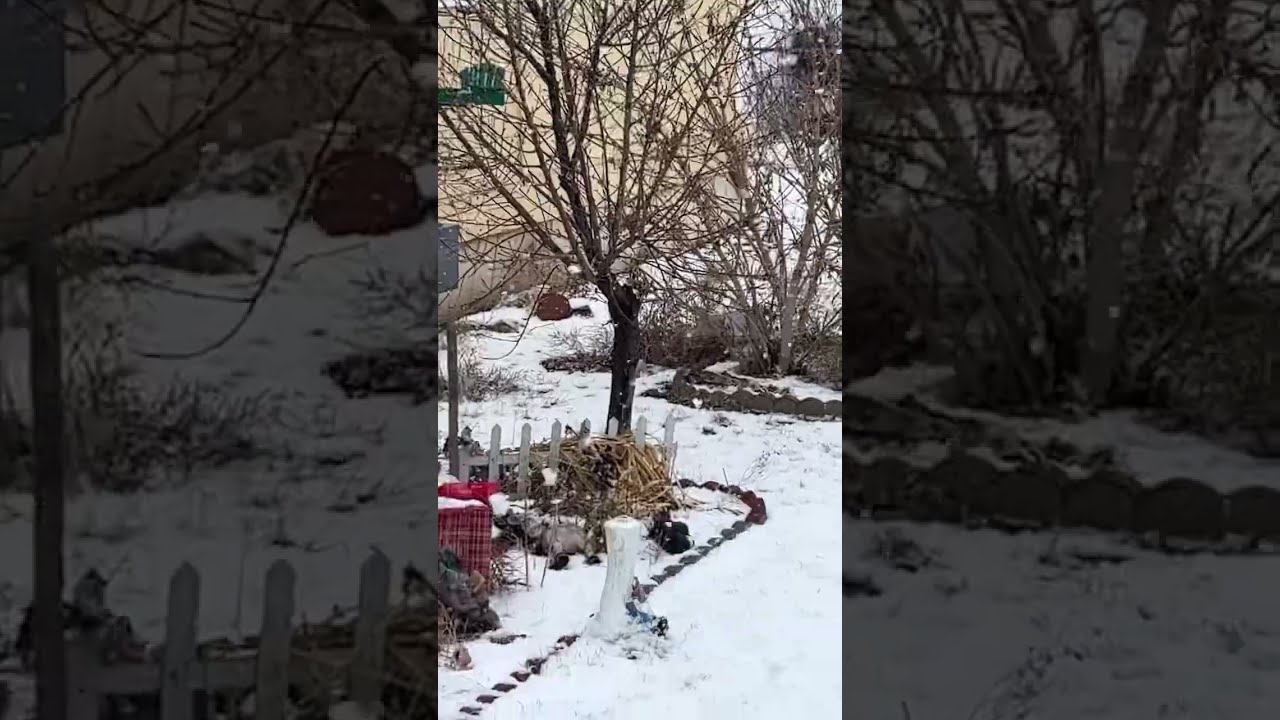This high-definition photograph is divided into three sections, with the central panel being the main focus. The image depicts a snow-covered suburban garden. In the center section, which is taller than it is wide, we see a tree surrounded by a border of small black rocks or bricks. A white picket fence stands behind the tree, and there is also a white tree stump and a red, multi-striped box—possibly a present—located to the right. Branches without leaves rest against the fence, contributing to the wintery atmosphere. In the background, tall brown trees with barren branches are visible alongside what appears to be a tall, tan-colored building. Further back, a grayish fence wraps around what looks like the bottom edge of a hill. The left and right sections of the photograph are close-ups that are blurred and semi-transparent, fading out to maintain the focus on the central snowy garden scene. The left inset shows a close-up of the white picket fence, while the right inset displays rocks and a bit of the road. The entire setup creates a serene, wintry tableau with an emphasis on the middle section, enhancing its smartphone-like shape.